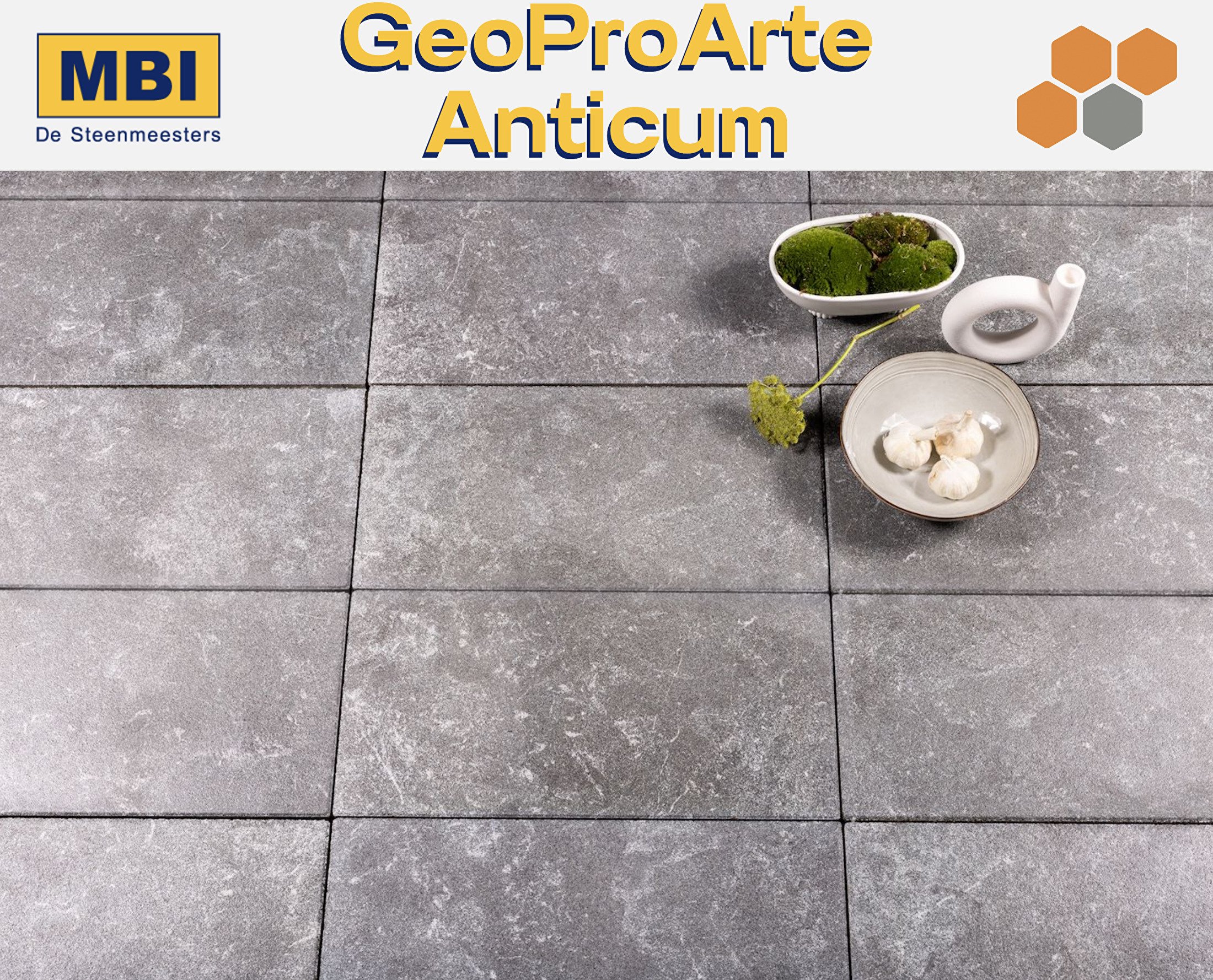This image is an advertisement displaying a smooth, rectangular stone flooring with small gaps between the tiles, accented by various shades of gray and sporadic white lines and splashes. At the top, a white banner features a yellow box with blue text reading "MBI De Steenmeesters" and "GeoPro Arte Anticum" in yellow text, accompanied by an orange and blue logo. In the top right corner, several objects are neatly arranged: two plates and a sauce dispenser. One of the plates is a tanned gray bowl containing three whole garlic bulbs. Beside it, there is an oval-shaped bowl filled with green moss-colored plants. Positioned between these dishes is a circular picture and green plant, contributing to the overall aesthetic of the setting. The colors in the image are predominantly blue, yellow, white, orange, gray, and green, harmoniously blending to create a visually appealing layout.